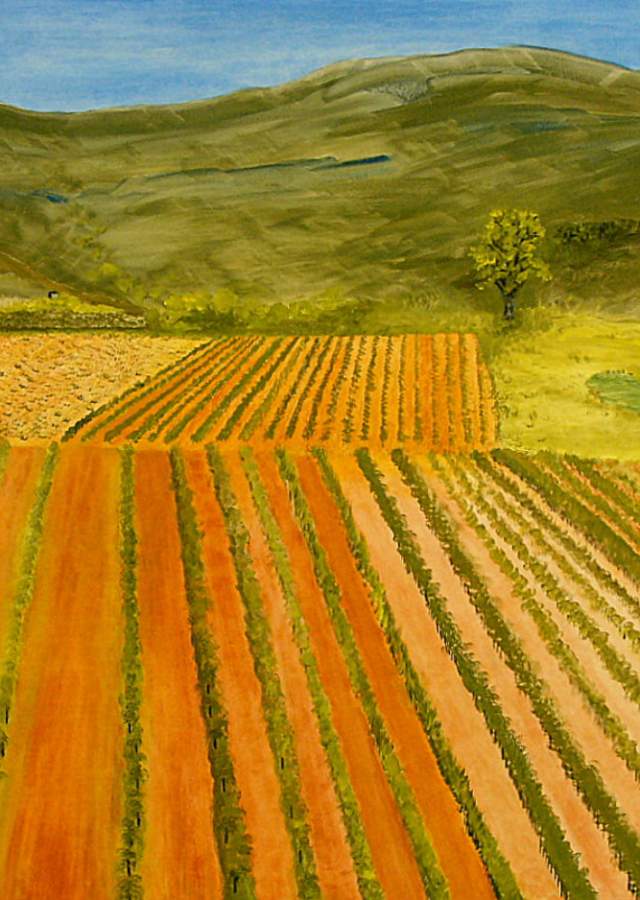The painting depicts a picturesque plot of farmland, dominated by vivid shades of green, orange-yellow, and blue. The composition showcases an undulating landscape of green hills under a blue, rolling sky. The fields are meticulously cultivated, presenting long, thin rows of green crops which are organized in square and rectangular patterns, suggesting an intentional agricultural arrangement. The ground is a rich brown hue interspersed with light beige strips of dirt, further highlighting the meticulous farming practice. At the base of the hills stands a small, vibrant green tree, its bright leaves providing a focal contrast against the cultivated land. The scene evokes a sense of structured, yet natural beauty, capturing the essence of rural farmland under a serene sky.